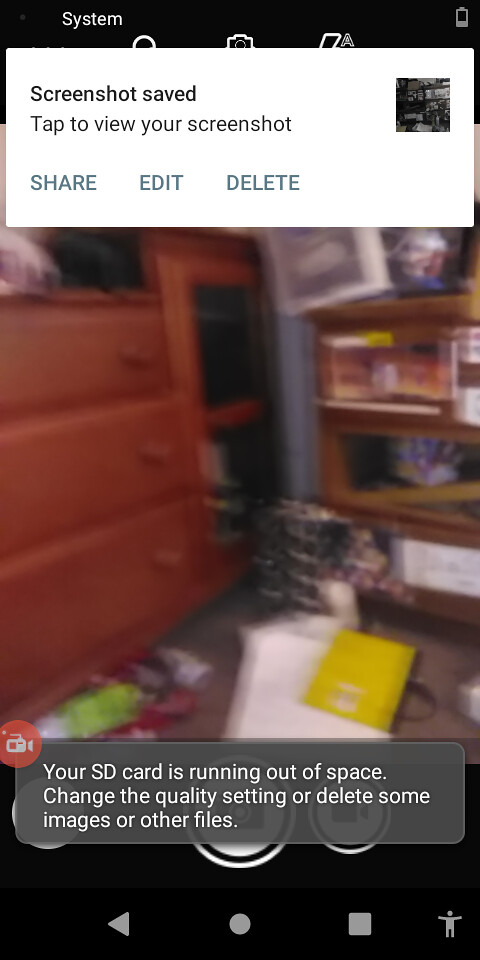This is a very blurry screenshot of a video capture taken on a phone, showing a disorganized bedroom. The screen displays a black bar across the top with a low battery icon and three other partially obstructed icons hidden by a white rectangular notification box that reads, "Screenshot saved. Tap to view your screenshot. Share, edit, or delete." In the inset blurry image, the bedroom features a wooden dresser with three long drawers on the left-hand side and a bookcase with three shelves on the right. There is a door in the back corner of the room, and various items like notebooks are scattered on the floor. At the bottom of the screen, another notification states, "Your SD card is running out of space. Change the quality setting or delete some images or other files," accompanied by three icons, including a video camera symbol. The bottom also displays standard control buttons such as stop, play, and record.